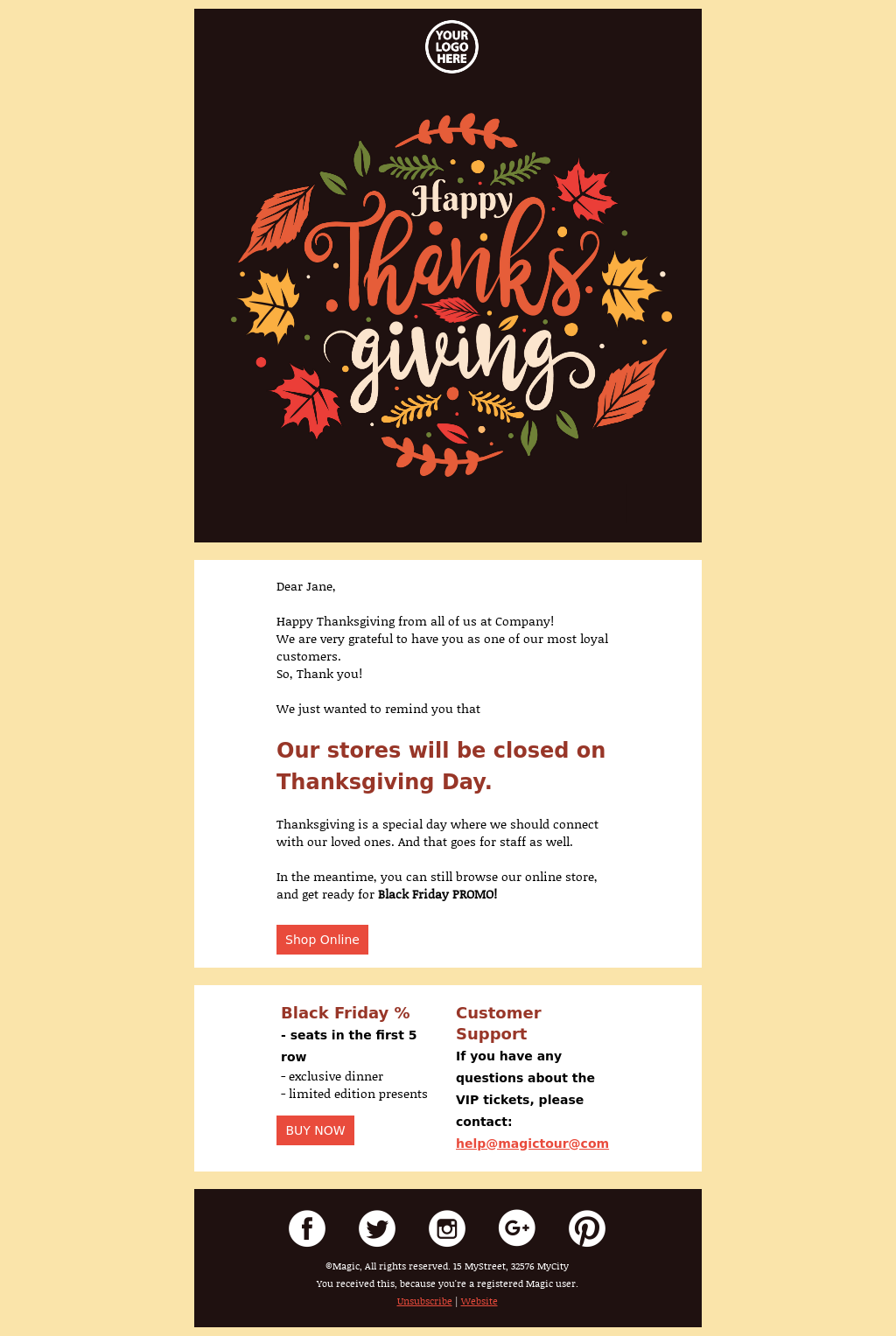This is a screenshot of a mobile-optimized website template featuring an autumnal and festive theme. The webpage is tall and rectangular, using a color palette reminiscent of Thanksgiving, with shades of tan, yellow, orange, red, and green. At the very top, there is a square banner with a dark brown background that displays placeholder text reading "Your Logo Here." Below this banner is an artistically designed wreath, adorned with yellow and red leaves as well as green twigs, and containing the message "Happy Thanksgiving" in the center.

Further down the page, a personalized message reads: "Dear Jane, Happy Thanksgiving from all of us at [Company]. We are very grateful to have you as one of our most loyal customers. Thank you." This area mimics a typical customer appreciation note and reflects the template's purpose of showcasing possible content.

Overall, this webpage serves as an example within a website builder, demonstrating what a completed Thanksgiving-themed page might look like once users customize it with their own logo and content.